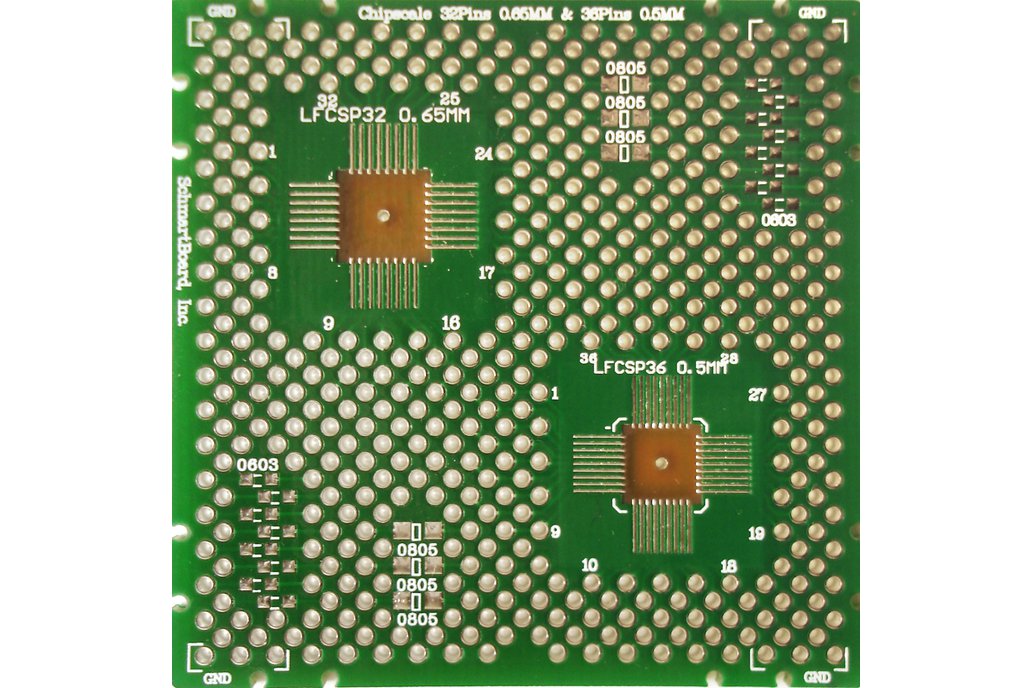The image depicts a detailed view of a green computer chip with a bright green surface. The chip is densely covered with white, silver, and gold balls, which may vary in color due to lighting. There are two prominent brown squares—one in the top-left and the other in the bottom-right quadrants. Each brown square features a central gold or silver ball and is surrounded on all four sides by gold bars or lines, with approximately seven parallel lines extending horizontally from each side. The surface also contains intricate white lettering and numbers, including "LFCSP320.65mm" in the top-left quadrant and "LFCSP360.5mm" in the bottom-right. Additionally, there are horizontal arrays of small, fuse-like components in the upper-right and lower-left quadrants, next to repeated sequences of the number "805." The meticulous detailing and complex patterning give the chip an advanced, technical appearance, reminiscent of intricate electronic circuitry.